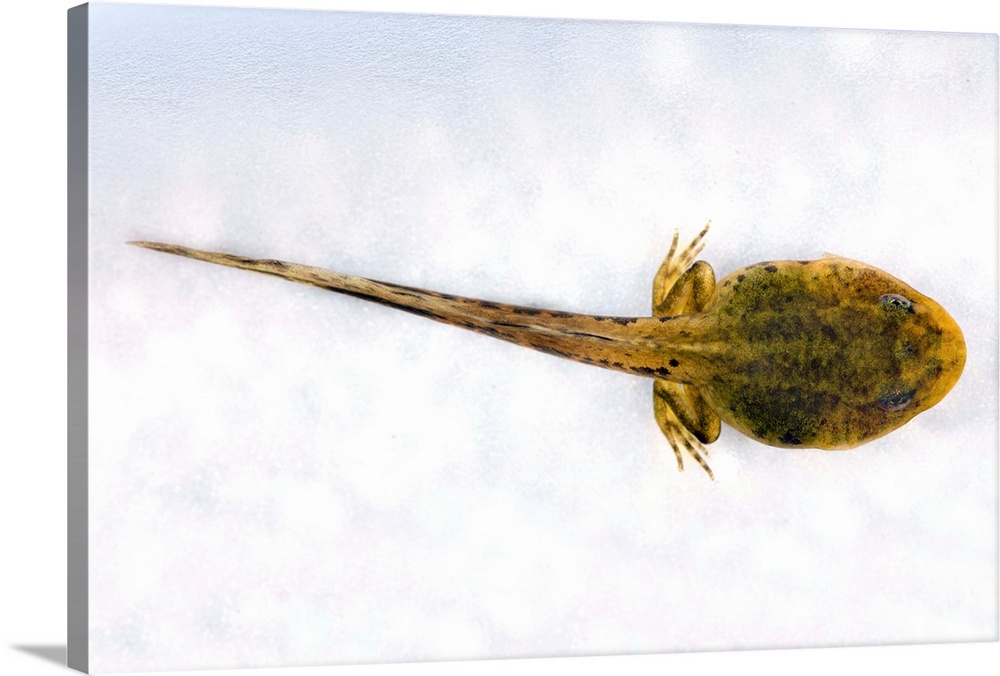This is an overhead, full-color painting of an evolving tadpole transforming into a frog, set against a mottled blue and white background. The tadpole's body stretches across a square canvas from the right side towards the left. Its head is lemon-shaped and faces the right side of the image, with striking black eyes. The creature is primarily green, featuring darker and lighter green tones with some brown and black spots peppered throughout its body. Its hind legs are partially developed, visible with toes, while its front legs have not yet emerged. A long tail extends from the center of its body to the left side of the canvas, with subtle black accentuating the outer edges and more splashes of brown and yellow. The background has some areas of white and light gray, providing a contrasting backdrop that enhances the vibrant colors of the tadpole.